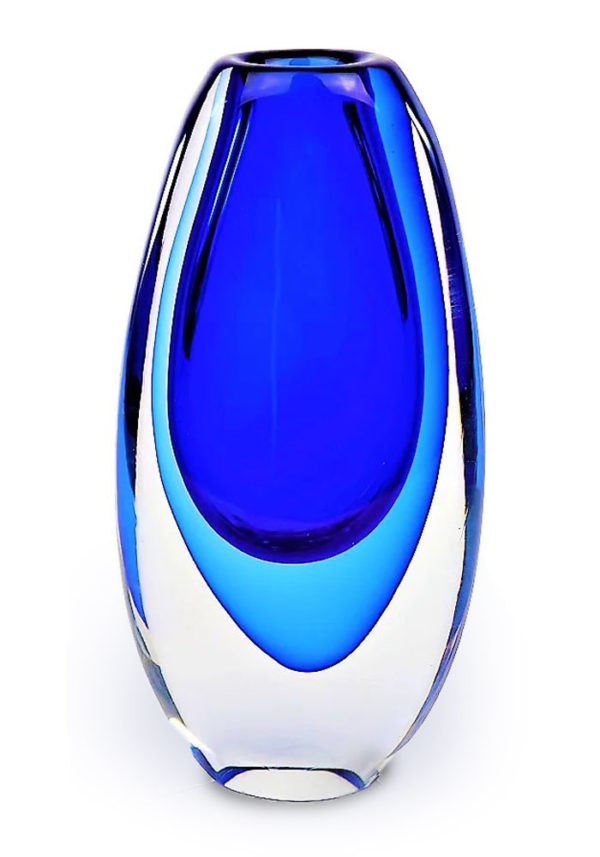The image depicts a tall, cylindrical vase, approximately 15-16 inches in height, crafted from clear glass on the exterior. The interior features a captivating gradient of blue hues: a darker blue at the center, transitioning to a lighter blue that forms a perimeter around it. The vase has a distinctive tiered design, with three levels; the top level is clear glass, followed by a lighter blue section, and finally the darker blue base. It creates a striking visual effect, almost resembling a layered jewel. A small, round opening at the top is designed for placing flowers or water. The vase stands alone in the image, with no additional context or background details provided.